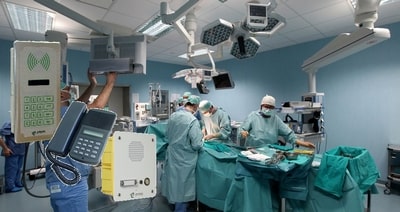This color photograph captures a busy hospital operating theater in landscape mode. The image, taken from a distance, showcases the entire suite, which features blue walls and a white ceiling. In the center of the room, seven health workers, some in green scrubs and others in blue, are engrossed in a surgical procedure. Four or five of these individuals, dressed in green gowns and caps, actively engage in the surgery, while the supporting staff in blue scrubs stand a few feet away, focusing on their respective tasks or adjusting equipment on screens. 

The operating table is draped in a light green sheet, matching the outfits of the primary surgical team. Bright surgical lights and several monitors, which descend from the ceiling on articulated arms, illuminate the scene. Rolling tables with medical equipment are strategically placed around the operating area. The patient, although central to the action, remains out of sight beneath the green drapery. 

In the bottom left corner of the photograph, somewhat incongruously, a black console-style telephone and a wall-mounted intercom system are superimposed atop the image. The yellow intercom box with its white cover, speaker, and various dials provides a touch of technological juxtaposition in this detailed snapshot of a modern surgical environment.